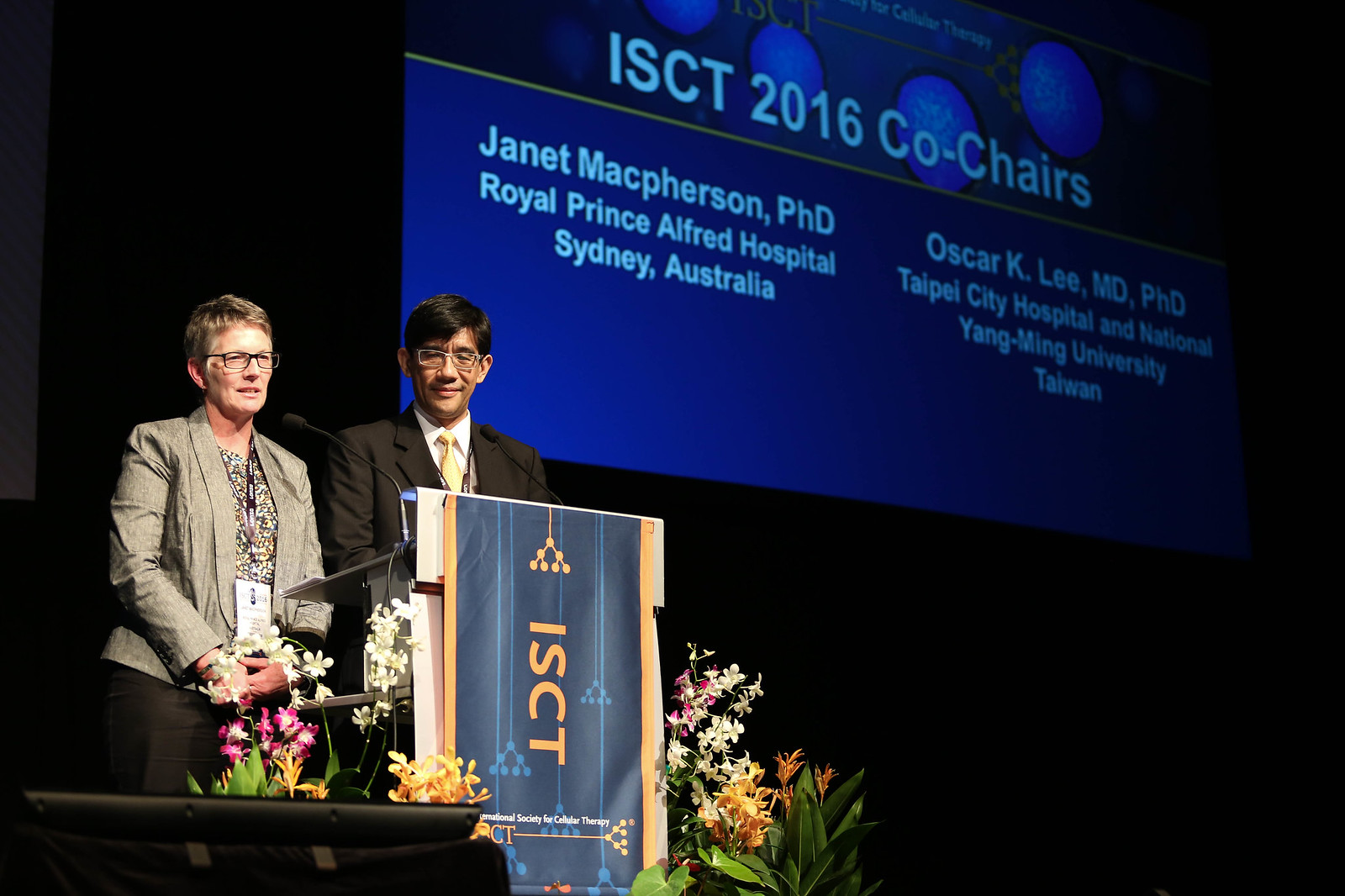This photographic image captures an indoor scene at a conference or award ceremony set in a hall. At the center of the image, a man and a woman are standing behind a podium adorned with a vertical ISCT banner. The podium is surrounded by an arrangement of flowers, adding a touch of elegance to the setting. Both individuals are wearing lanyards, and each is equipped with eyeglasses.

The man, appearing to be of Asian descent and likely in his 40s, is dressed in a dark suit with a yellow tie and a white shirt. He has dark hair and is seen looking downward. The woman, on the other hand, has lightish red hair and wears a greyish-brown jacket over a brown and white blouse. Both individuals are formally dressed, indicating the event's professional nature.

Above and to the right of the podium, a slide projected on a screen reads, "ISCT 2016 Co-Chairs." It lists the names and affiliations of the two individuals: Janet McPherson, Ph.D., from Royal Prince Alfred Hospital, Sydney, Australia, and Oscar K. Lee, M.D., Ph.D., from Taipei City Hospital and National Yangming University, Taiwan. This suggests that Janet and Oscar are the co-chairs of the event, and their poised demeanor implies they might be in the midst of delivering a presentation or addressing the audience.